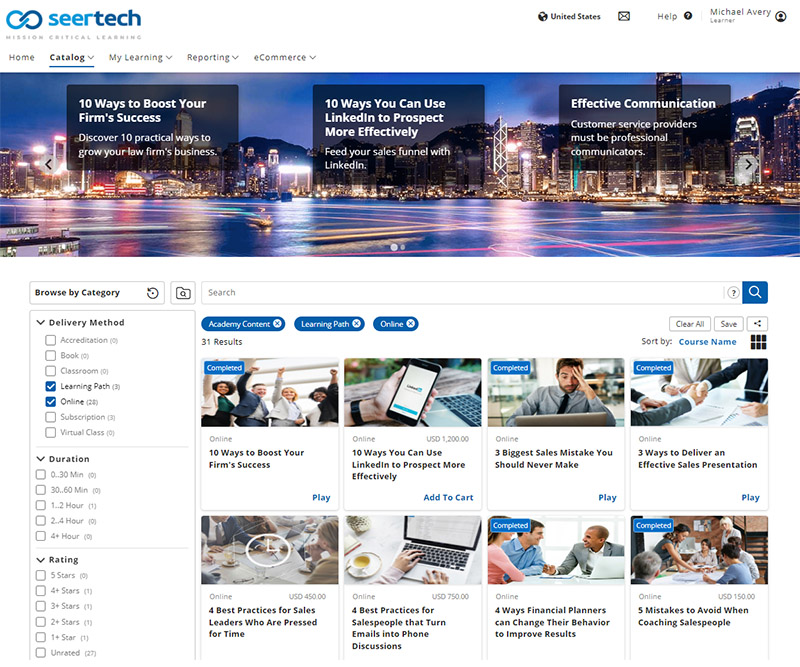This image showcases a webpage from a business consulting or productivity website named SeerTech. In the top left corner, there's a distinctive logo featuring an infinity symbol, with the left side of the infinity in a lighter blue and the right side in a darker blue. Adjacent to the logo, the name "SeerTech" is displayed in matching colors - the word "Seer" in a lighter blue, and "Tech" in a darker blue.

The banner of the webpage prominently features a semi-transparent black box overlaying a nighttime cityscape. This section is designed to capture attention with bold text stating, "10 Ways to Boost Your Firm's Success," accompanied by a sub-heading, "Discover 10 practical ways to grow your firm's business." Additional highlighted articles on the banner include "10 Ways You Could Use LinkedIn to Prospect More Effectively" and an insight into maintaining "Effective Communication" for customer service providers to enhance professional interactions.

On the left-hand side of the page, there's a categorized list, organized into approximately 15 different topics. Each category appears to be broken down by delivery method, duration, and rating.

To the right, several tags such as "Academy," "Content," "Landing Pads," and "Online" are displayed, each with a white X next to them likely indicating the option to remove or filter by these tags. Nearby, a share button is present, facilitating easy sharing of the content.

Below the banner are eight learning modules, each represented by square thumbnails featuring various images related to collaboration. The titles of these modules are written in black text beneath each corresponding image, emphasizing different facets of business productivity and skills development.